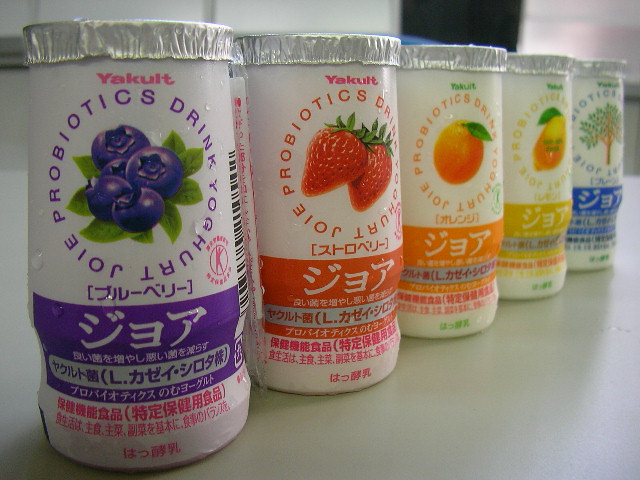This photograph features five yogurt drink cups, prominently displayed in a row on a smooth surface with a white to gray gradient. The cups, which are designed to resemble narrow soda cans, each feature a foil top crimped around their edges and a distinct vibrant label. Starting from the left, the first cup is highly prominent, filling the entire height of the frame. This cup features a purple label adorned with images of purple berries, showcasing the product's flavor. The text on the label reads "Probiotics Drink Yogurt Joy," and is accompanied by white Japanese characters. 

As the line of cups progresses to the right, each subsequent cup recedes slightly into the background, creating a visually appealing diagonal arrangement. The second cup has an orange label with a strawberry motif, while the third, also orange in color, depicts an orange fruit. The fourth cup sports a yellow label with lemon imagery, and the final cup, somewhat blurred due to the depth of field, has a blue label with the image of a tree.

All the cups bear a pink logo at the top reading "Eocult" on the first two, with the remaining three cups featuring the logo in green. Near their bases, the cups have indentures designed for an easier grip. The perspective of the image makes the cups appear to decrease in size as they recede into the background, sitting on a gray counter with a white backdrop, adding depth and dimension to the composition.